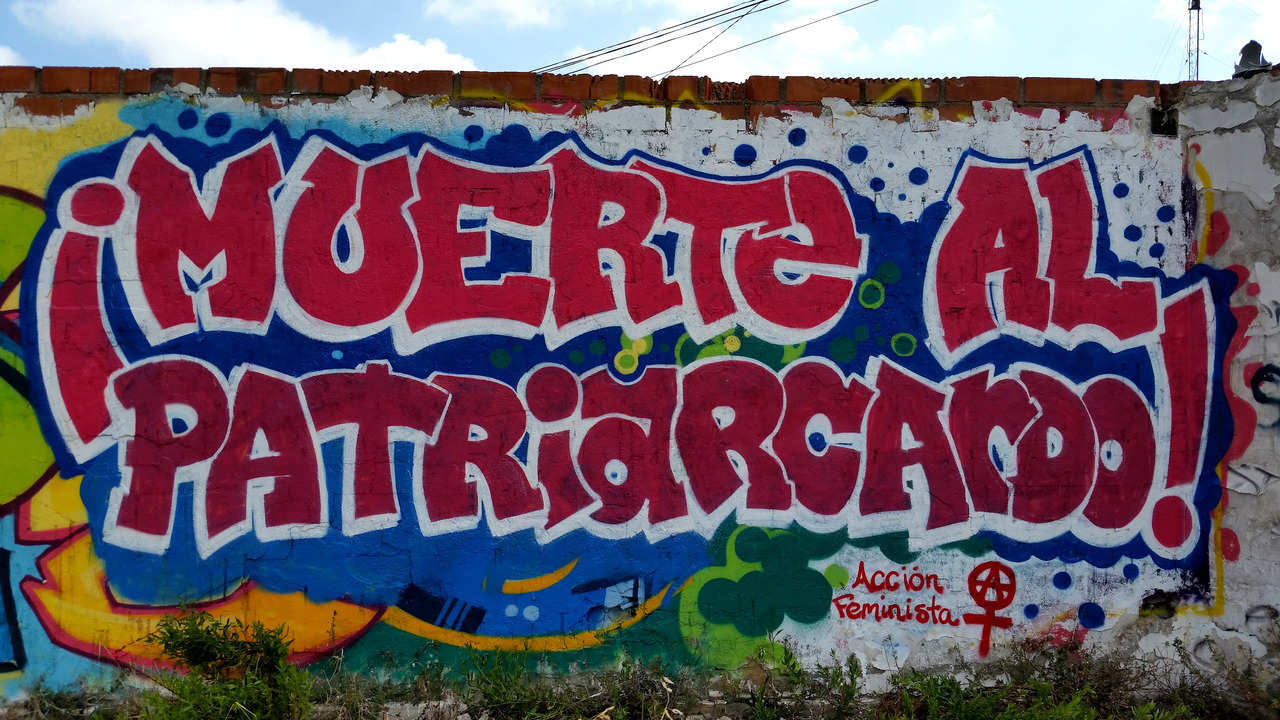In this vibrant image, a graffiti-covered wall bursts with an array of colors and dynamic designs. The wall features inscriptions such as "Aymwete Al," "Patriarca 2," and "Asensación Feminista," contributing to its eclectic and thought-provoking aesthetic. Above the graffiti, a network of electric lines crisscrosses, adding an urban element to the scene. In the top right corner, a mask—possibly representing a network—can be seen. The backdrop of the image reveals a bright, clear day with scattered clouds, suggesting a crisp and cool atmosphere. The color palette of the graffiti is notably diverse, featuring bold hues of red, blue, orange, yellow, green, and white, making the artwork a captivating focal point against the urban landscape.